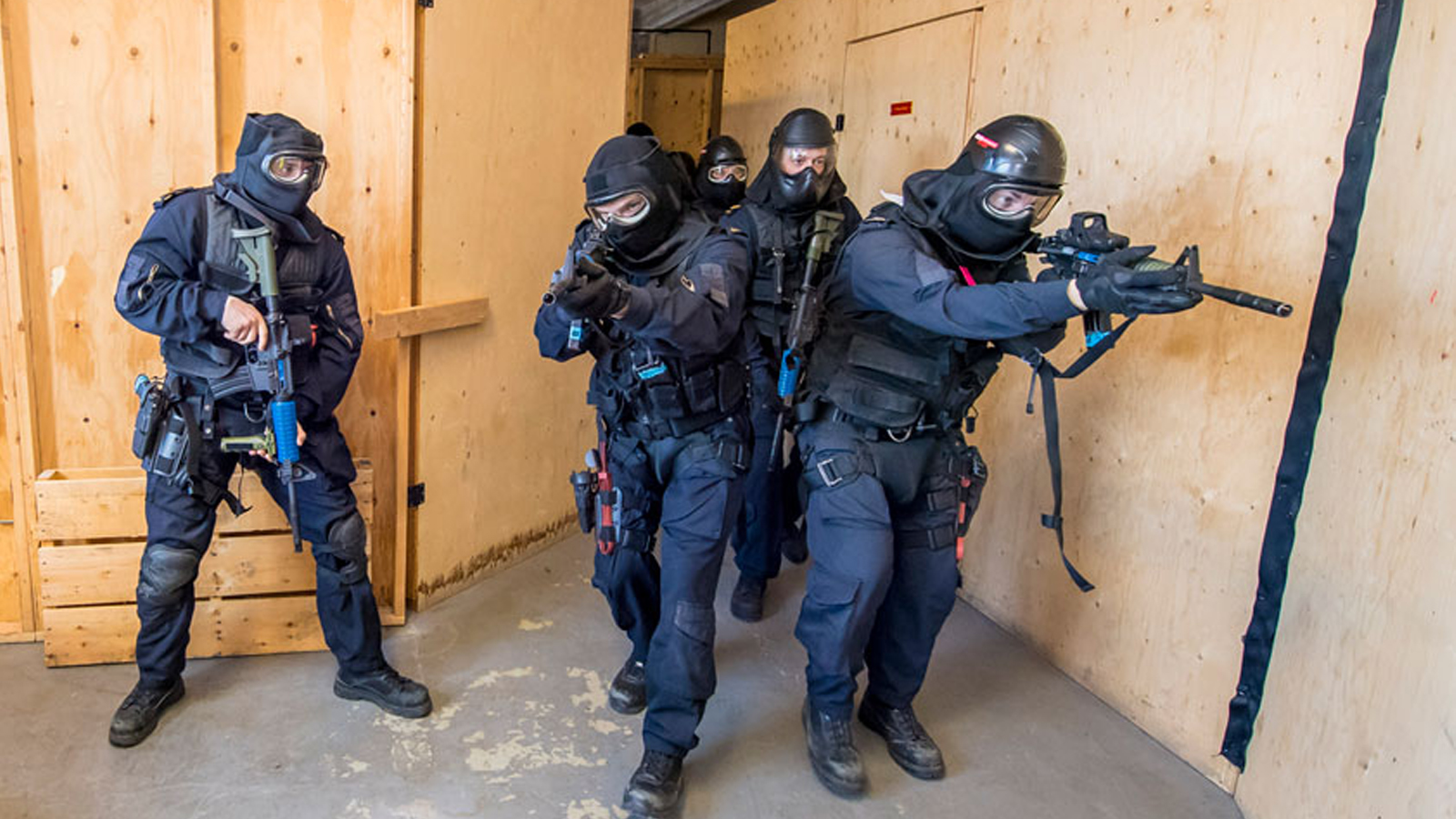This color photograph captures a group of SWAT team members, identifiable by their police uniforms and tactical gear. The uniforms are primarily blue, complemented by black bulletproof vests, black boots, and sidearms secured in holsters. Each officer is equipped with a helmet and goggles, and they are holding rifles, specifically combat rifles. The scene is set within an unfinished room with bare plywood walls and a gray concrete floor, partially worn with exposed cream patches. The setting includes a cut-out doorway in the plywood and a half pallet visible behind one of the men. In formation, three officers stand prominently in the foreground; the two officers on the right have their rifles pointed ahead, while the officer to their left points his rifle downward. Additional officers are seen lining up in the background, advancing through a hallway. Their faces are obscured by masks, reinforcing their readiness for tactical action.